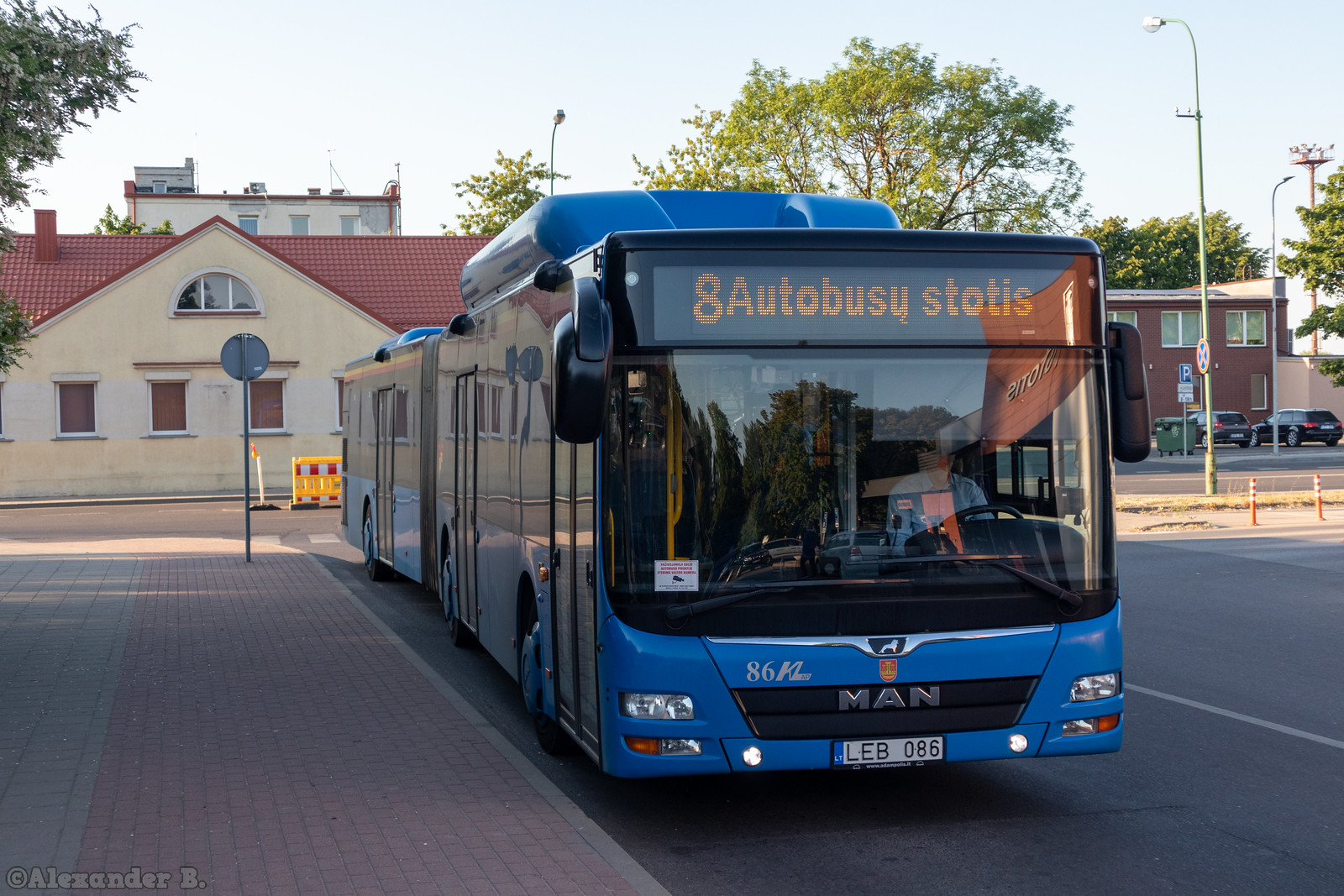The outdoor image features a modern blue passenger bus parked on a paved, brick-tiled sidewalk. Prominently displayed in lights across the top of the bus are the words "8 auto bussy." The bus's front window has a glare, obstructing a clear view inside, but a driver in a blue jacket and possibly an orange or pink shirt can be seen seated at the steering wheel. The bus's front is marked with clear headlights and a license plate reading LEB086. 

In the backdrop, there's a large house with a light beige color and a brownish-red roof, adorned with multiple windows, including a distinctive circular or half-circle window on the top. Adjacent to this is another white house featuring white window frames. The scene is enriched with tall green trees and additional structures, including a building with a parking lot in view and several parked cars.

The setting includes white street lamps and a street sign turned away, making it unreadable. The road is paved and marked with white lines, adding to the structured urban environment.